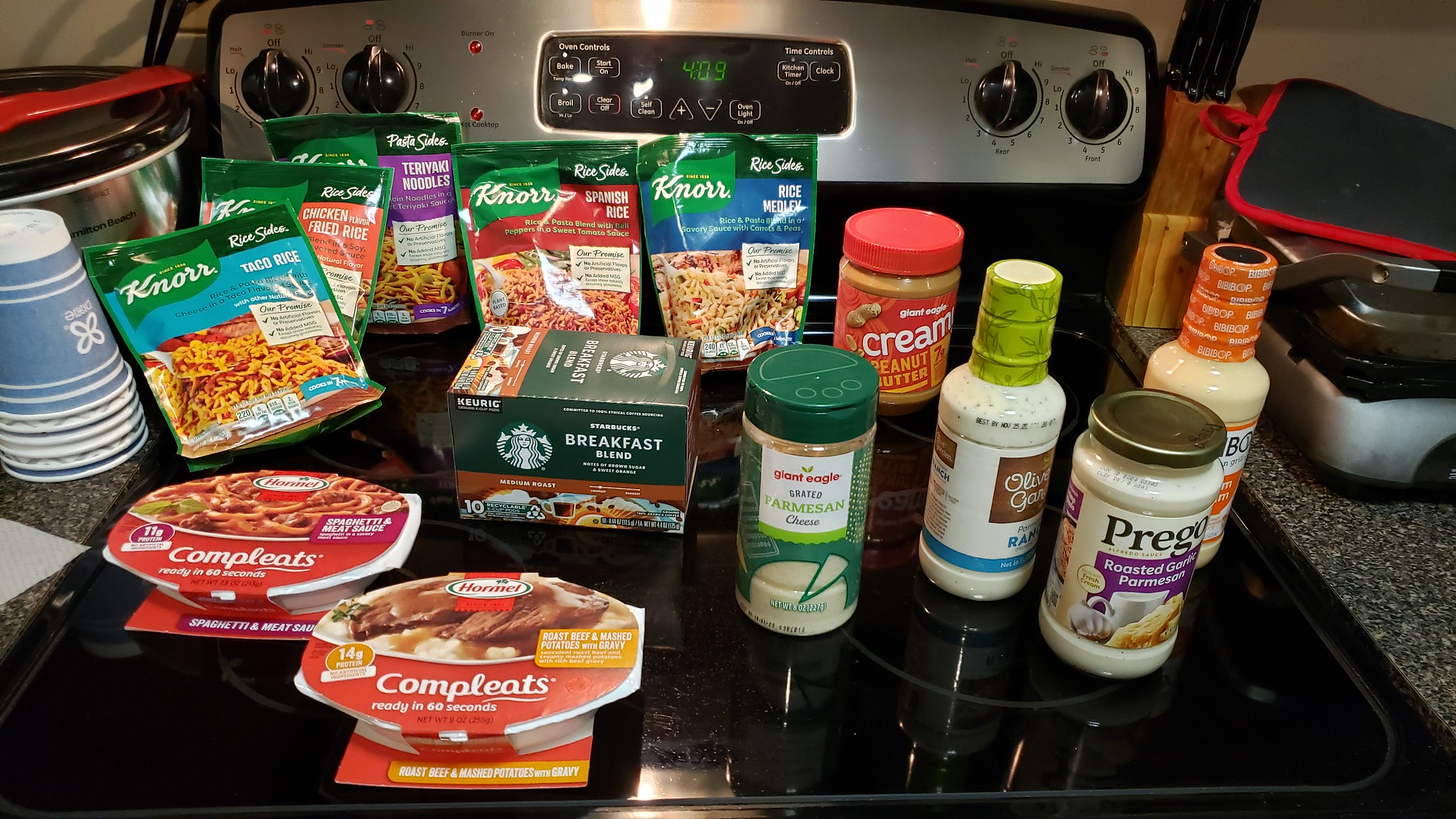The image is a detailed rectangular landscape photograph of a modern kitchen stovetop, predominantly black with a sleek silver back panel. The smooth, flat-top range features four burners, flanked by two black knobs on each side of the central digital display that reads “4:09” in green. Arranged atop the stove are an assortment of convenience foods and groceries, meticulously detailed as follows: 

- **In the center**: Several packets of Knorr instant rice and pasta, including Taco Rice, Rice Medley, Spanish Rice, Fried Rice, and Teriyaki Noodles, leaning against the back panel.
- **Towards the right**: A glass bottle of Prego Roasted Garlic Parmesan Sauce, a bottle of Olive Garden Ranch Dressing, a jar of Giant Eagle generic creamy peanut butter, and another unidentified plastic bottle with an orange lid. 
- **In the lower center**: A green container of grated Parmesan cheese from Giant Eagle.
- **To the left of center**: A box of Starbucks Breakfast Blend Keurig coffee.
- **In the lower left**: Two packs of Hormel Completes—Spaghetti with Meat Sauce and Roast Beef with Seasoned Potatoes. 

Adjacent to the stovetop:
- **To the left**: An upside-down stack of six to seven paper cups.
- **In the upper right corner**: What appears to be a closed panini press. 

This curated collection of convenience foods covers the black stovetop, framed by a granite-looking countertop on either side, ready to be used for meal preparation.